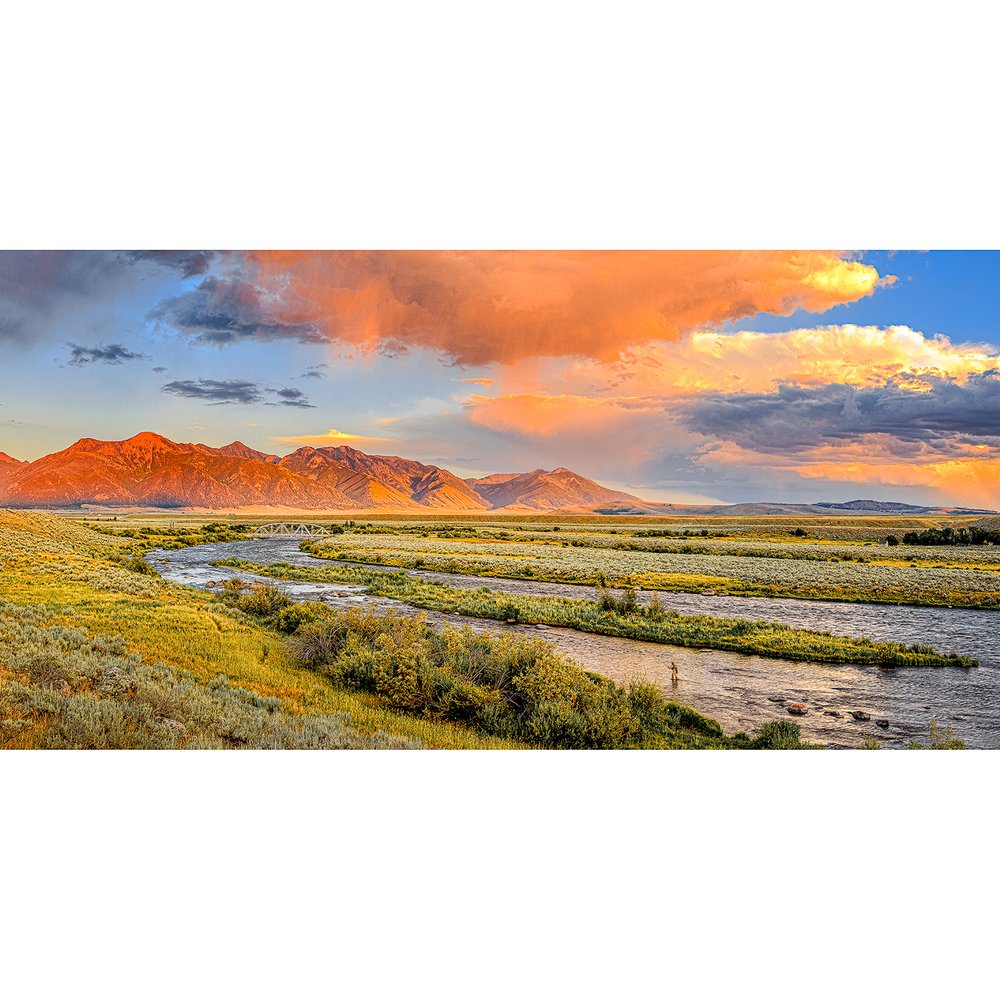This visually striking image, likely a painting, captures an idyllic outdoor scene during what appears to be either sunrise or sunset, imbuing the landscape with rich, warm tones. Horizontally rectangular in format, the scene unfolds under a sky awash with hues of blue, orange, and yellow. Billowing clouds, varying in shades of white, gray, and orange, drift across the sky, adding to the surreal ambiance.

The scene is dominated by a rugged mountain range positioned off-center to the left. These mountains have sharp, jagged peaks and appear brown or even grayish rock, devoid of snow. Patches of green foliage pepper the lower slopes, contributing to the visual richness. In front of these mountains stretches a grassy field dotted with patches of vibrant, small yellow flowers.

At the lower portion of the image, a serene body of water reflects the orange tint of the sky, suggesting a tranquil river or stream. This central water body could be a large, meandering rice paddy, hosting long strips of fertile land. Around and within the water, lush grassy fields and small islands are interspersed, each adorned with a mix of green grass and numerous white flowers.

In the far distance, a white metal suspension bridge spans the river, subtly integrated into the landscape. This delicate human element complements the untouched beauty of the natural surroundings, creating a harmonious blend of nature and subtle human presence. The overall scene, possibly semi-desert, evokes a sense of peace and timeless beauty, encapsulated in the soft interplay of light and shadow.